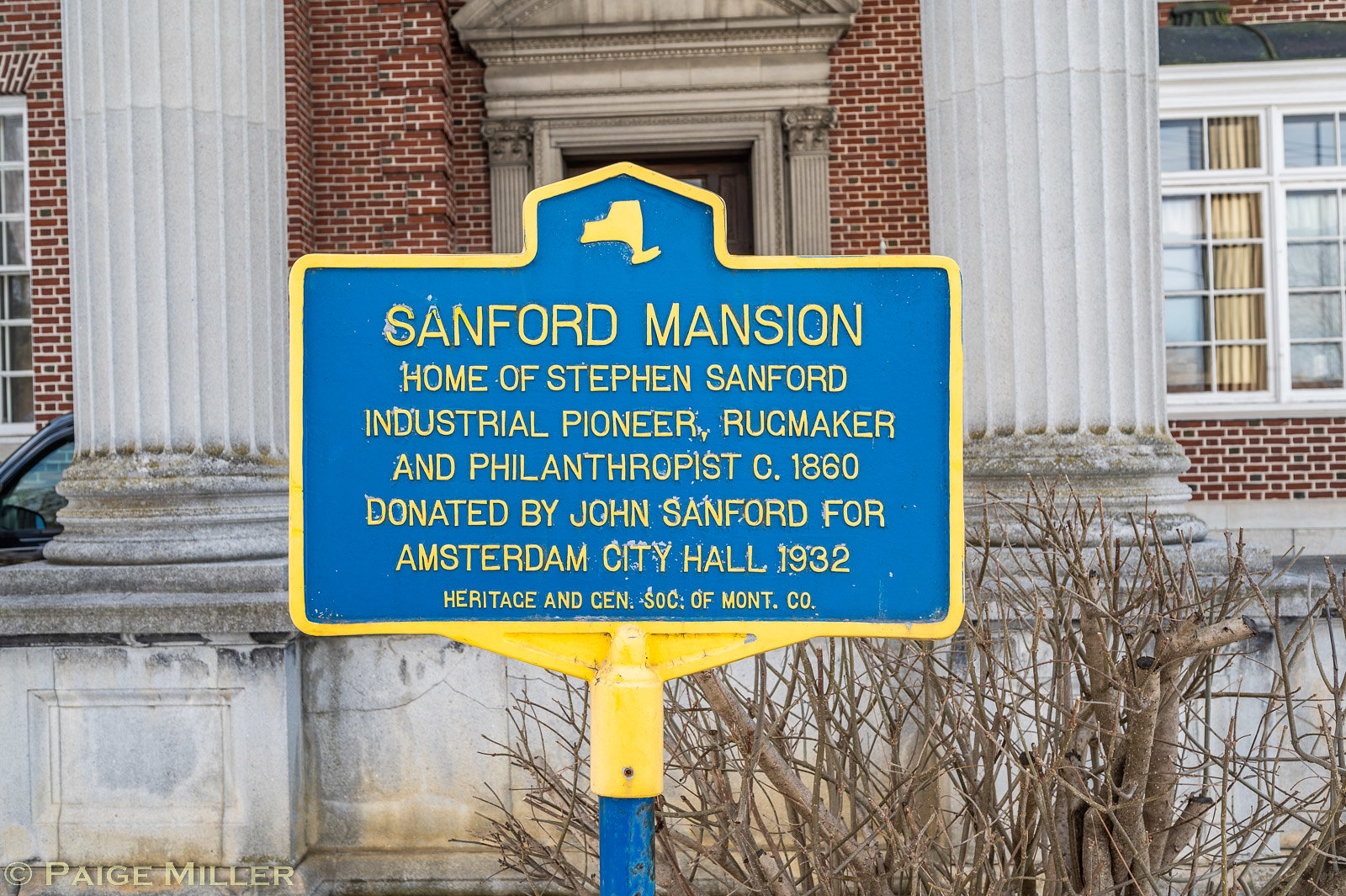The image is a colored daylight outdoor photograph showcasing a historic site. In the foreground, there is a prominent blue metal sign with a yellow outline and a silhouette of a house at the top, attached to a blue pole with a yellow border. The sign features yellow text that reads: "Sanford Mansion, Home of Stephen Sanford, Industrial Pioneer, Rugmaker, and Philanthropist, circa 1860. Donated by John Sanford for Amsterdam City Hall 1932. Heritage and Gen. Soc. of Montco." Below this, towards the bottom left of the sign, there is a watermark displaying a seed trademark icon with the text "PAIGE MILLER" in white. The background reveals a large red brick building with two large white stone pillars flanking a dark brown wooden door entryway. Additionally, the building has white grid-pattern windows. In the lower right corner, the photo captures the bare branches of a leafless bush. The overall shape of the photograph is rectangular, wider than it is tall.